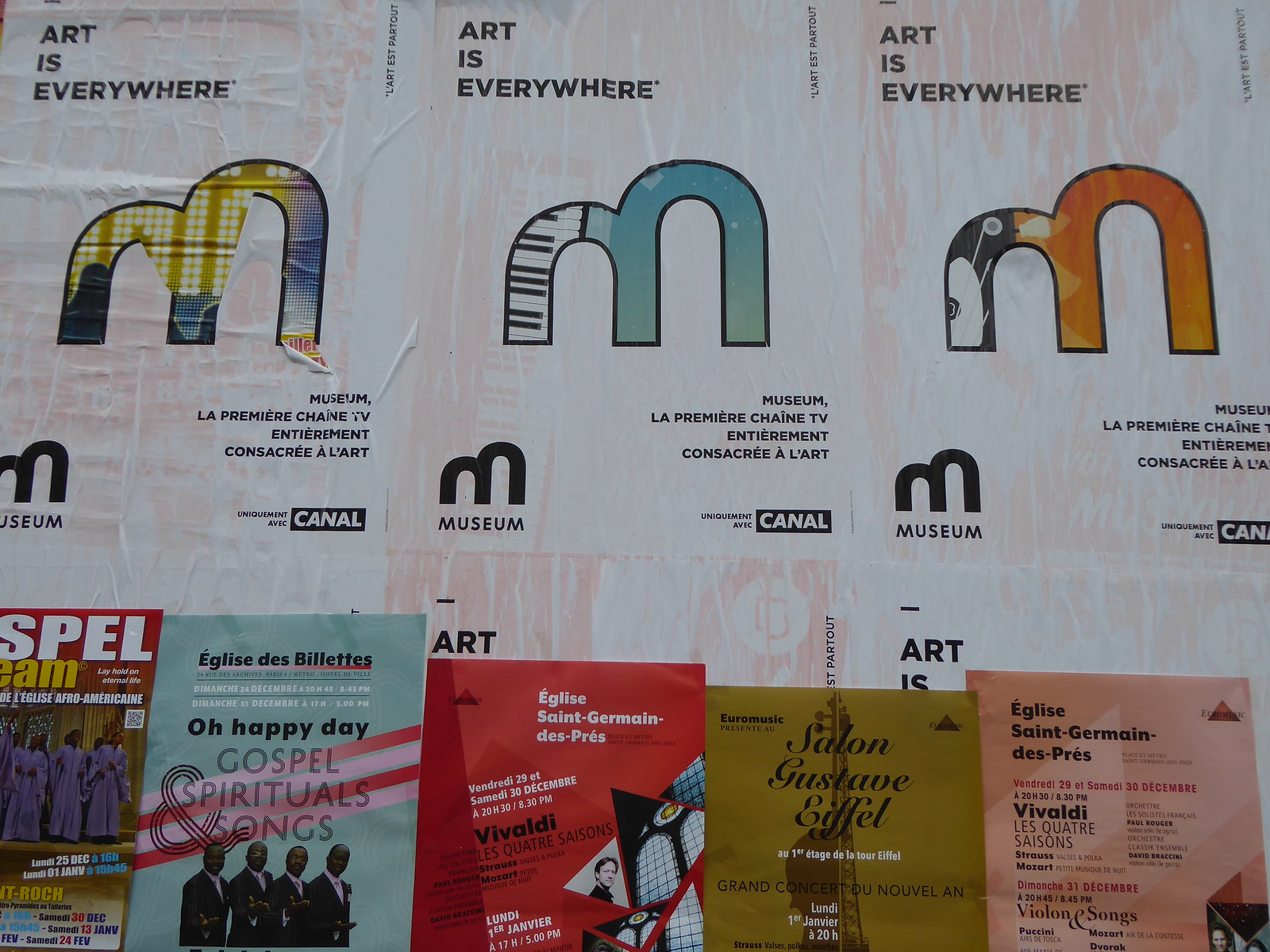In this detailed image, multiple elements combine to convey a vibrant and eclectic celebration of art and culture. Dominating the scene is a prominent poster in the background proclaiming "Art is Everywhere Museum," with dynamic, repetitive use of the letter "M" in various styles and positions, enhancing the visual appeal. Below the poster, a neat arrangement of five books lines the bottom of the image. These books display diverse titles such as "Gospels, Spirituals, and Songs," "Vivaldi," "Salon," and "Gustavi, Eiffel," reflecting a broad spectrum of artistic and cultural themes.

The color palette is rich and varied, featuring hues of white, black, pink, yellow, light blue, dark blue, orange, gray, red, tan, and purple, contributing to a lively and engaging visual experience. Intriguingly, there are also magazines in different colors, including red, green, and yellow, with one positioned in the bottom left corner showcasing the acronym "SPL" at its top. Partially obscured text on these magazines suggests elements in French, with one notably displaying a logo with the word "CANAL" spelled out.

Overall, the scene is set indoors and evokes the energetic atmosphere of an art show or festival, where a harmonious blend of books, posters, and magazines invites viewers to immerse themselves in the diverse world of art and culture.